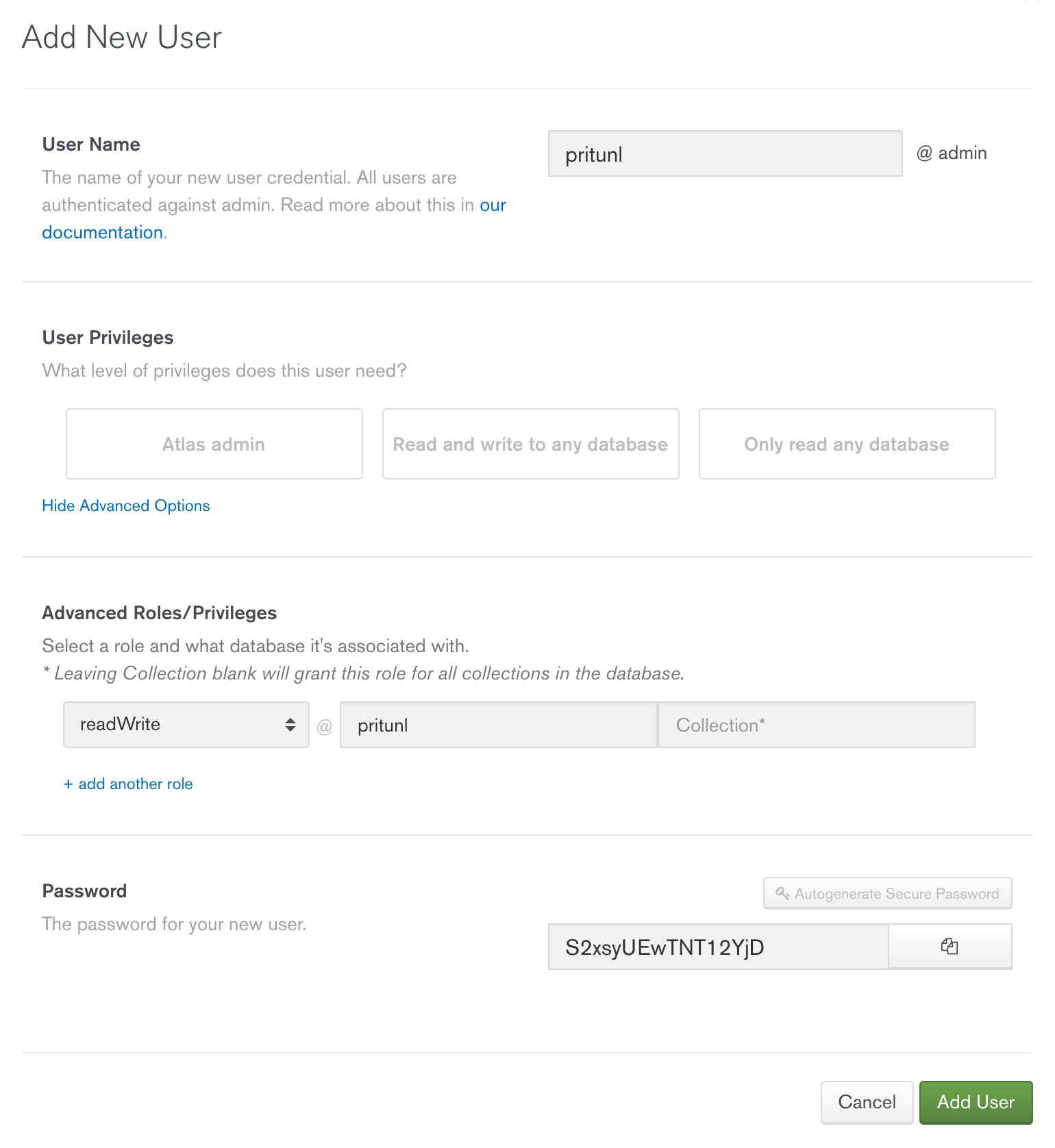At the top left, the interface displays an "Add New User" header, followed by a very thin, faint gray line. Below this line, the text "Username" is displayed in bold letters, indicating the field for entering the new user credential. All users are authenticated against the admin account, with a prompt to "Read more about this in our documentation," where "documentation" is highlighted in blue as a clickable link.

To the right, there's a gray text field with the letters "P-R-I-T-U-N-L" in bold, followed by an "@" symbol, and then the word "admin." Another faint gray line separates this section from the "User Privileges" area, where "User Privileges" is in bold text. Instructions ask what level of privileges the user needs, offering options such as "Atlas Admin," "Read and Write to any database," and "Read-only access to any database." 

Highlighted in blue, "Hide Advanced Options" appears below another faint gray line. This section references "Advanced Roles/Privileges" and includes a note in slanted text stating that "leaving collection blank will grant this role for all collections in the database." The role "Read Write" is followed by "P-R-I-T-U-N-L" and a text field for the collection, denoted with a star. A plus symbol next to the text "Add another role" is also highlighted in blue for adding additional roles or privileges.

Another gray line sets off the final section, marked "Password," which requires entering a password for the new user. An example, "AtS2XSYUEWTNT12YJT," is followed by options to "Auto Generate Secure Password" and a "Copy" button. At the bottom of the interface, the options "Cancel" and "Add User" are available for concluding the setup process.